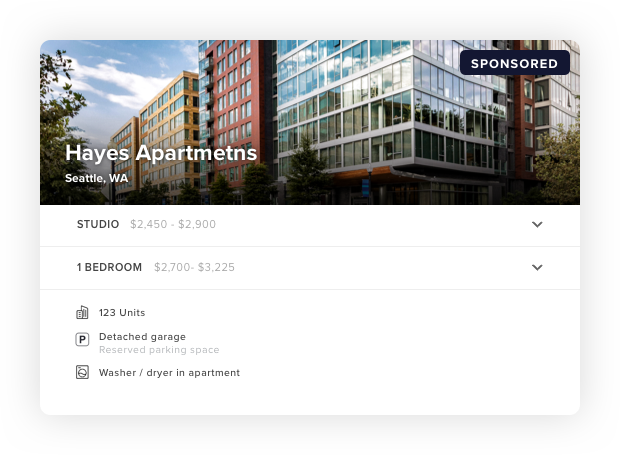The image is a detailed screenshot of a real estate listing for Hayes Apartments located in Seattle, Washington. At the top of the listing, there is an exterior photograph of the apartment complex. The listing provides two types of units: studio apartments, which range in price from $2,450 to $2,900, and one-bedroom apartments, which range from $2,700 to $3,225. The building comprises a total of 123 units. Amenities include a detached garage with reserved parking spaces and in-unit washer and dryer facilities.